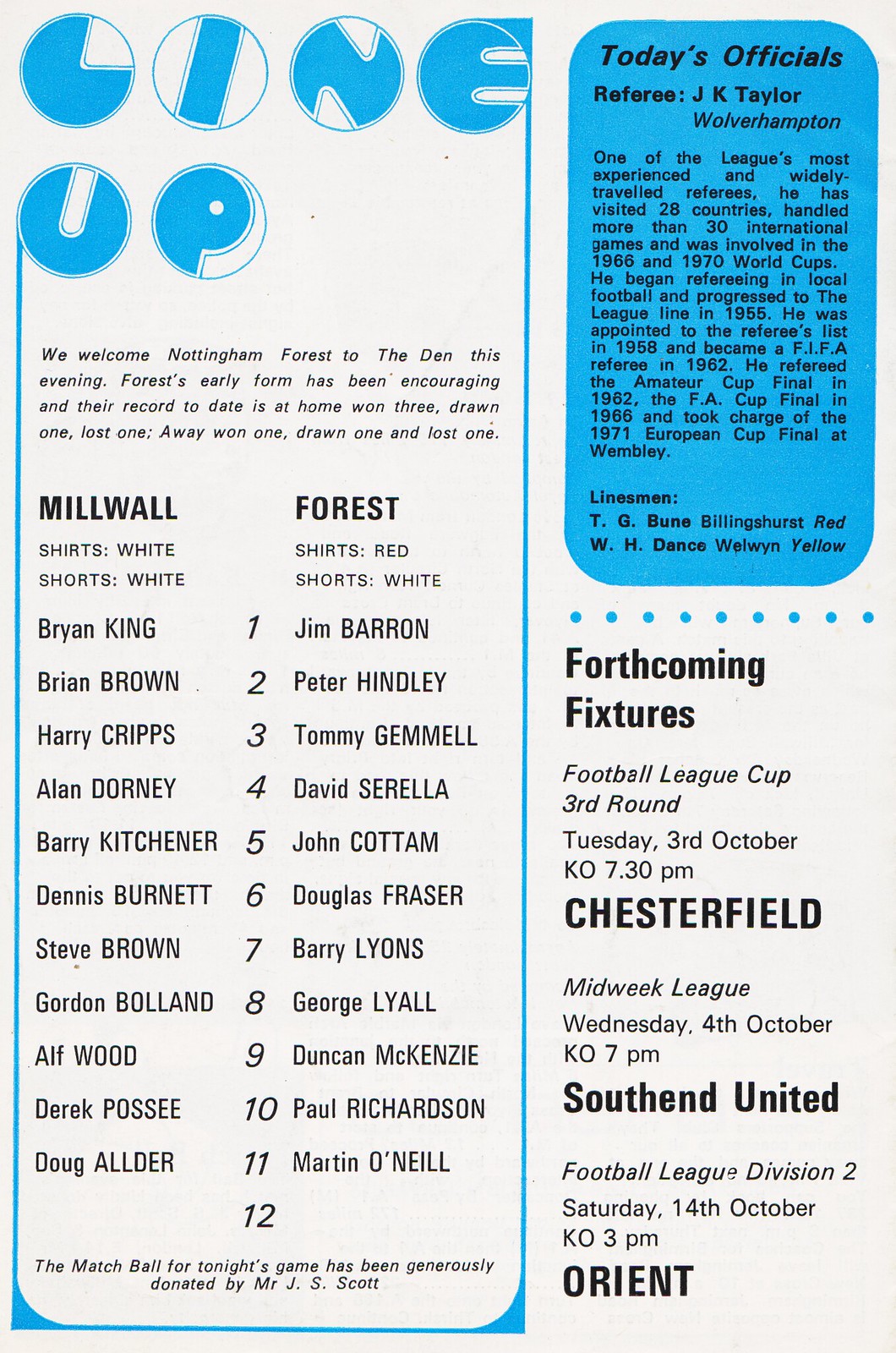The image displays a page from a sports periodical featuring a detailed breakdown of a football match lineup, officials, and forthcoming fixtures. Dominated by blue, white, and black hues, the page reveals a heading in graphic blue font on the left two-thirds labeled "Line Up," under which players are listed by number along with information about their jerseys. Millwall's lineup showcases their all-white kit — shirts and shorts — with players named: Brian King, Brian Brown, Harry Cripps, Alan Dorney, Barry Kitchener, Davis Burnett, Steve Brown, Gordon Boland, Al Floyd, Derek Posse, and Doug Adler. Nottingham Forest, the visiting team, will be clad in red shirts and white shorts, featuring players such as Jim Barron, Peter Henley, Tommy Gemmell, David Serella, John Cormen, Douglas Fraser, Barry Lyons, George Lyall, Duncan McKenzie, Paul Richardson, and Martin O'Neill.

The right-hand side of the page features a blue subsection "Today's Officials" in italic text, spotlighting Referee J.K. Taylorman from Wolverhampton, known for his extensive international experience, including officiating in the 1966 and 1970 World Cups. Linesmen T.G. Beun and W.H. Dance are also listed, with respective identifiers.

Beneath this, under the "Forthcoming Fixtures" heading in white text, are the upcoming matches: Chesterfield on Tuesday, October 3rd at 7:30 p.m., Southend United on Wednesday, October 4th at 7:00 p.m., and Orient on Saturday, October 14th at 3:00 p.m. The page also notes the welcoming of Nottingham Forest to "The Den" for the evening, mentioning their notable early season record.

Emphasis is given to the stark contrast of both teams' kits, the detailed listing of each team's player lineup, and the professionalism of the officiating personnel, rounding out a comprehensive and richly detailed sports page.